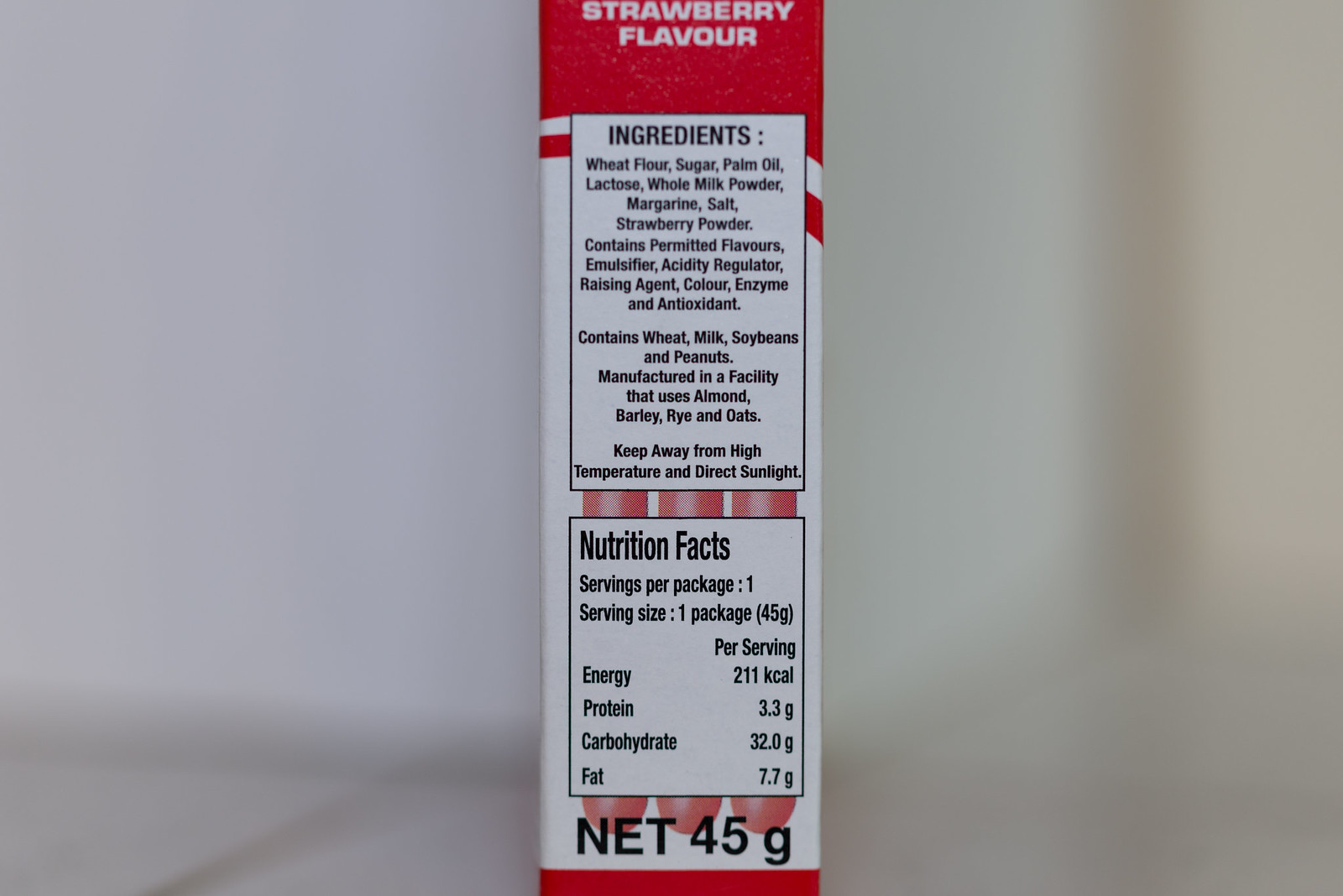The photograph depicts the side panel of a food packaging box, specifically a white carton with red trim. At the top of the side panel, the words "Strawberry Flavor" are prominently displayed in white text on a red background. Below this, there is a white box outlined with a black line that lists the ingredients in black text, including wheat flour, sugar, palm oil, lactose, whole milk powder, margarine, salt, strawberry powder, permitted flavors, an emulsifier, an acidity regulator, a raising agent, color, enzyme, and an antioxidant. Further down, another box provides the nutrition facts, indicating that the serving size is one package (45 grams). At the very bottom, in larger black letters, the net weight is clearly stated as "Net 45G." The entire side panel of this packaging is photographed against a plain white background.